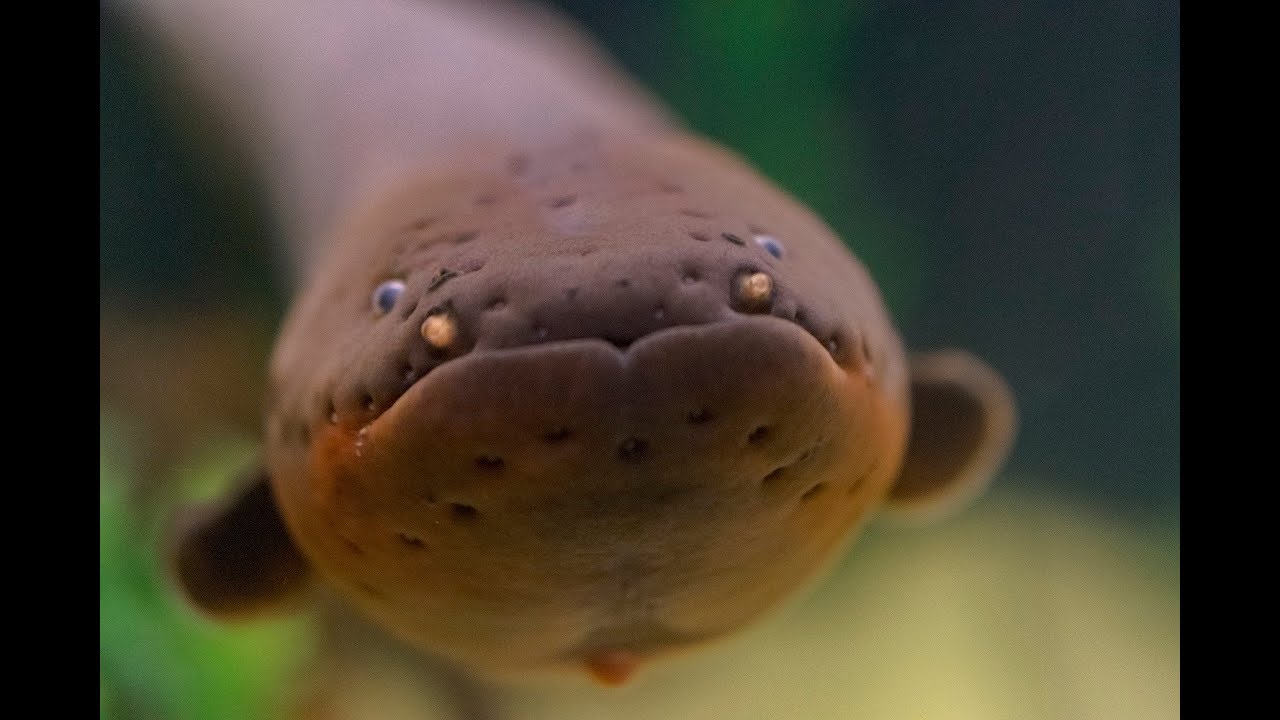This is a photorealistic landscape image of an eel, captured from a video as evidenced by the thick black borders on the left and right sides of the photo. The focus is on the eel's face, which is incredibly close to the camera and highly detailed. The eel's mouth is closed and pressed nearly up against the lens, making it the most prominent feature in the foreground. The eel has small white eyes with black pupils, and its face is adorned with two yellowish nostrils positioned above the mouth. The skin is brown, smooth, and covered in subtle pock marks, including small holes on its head and under its chin. Protruding from either side, there are fins that are out of focus due to the shallow depth of field. Additionally, an orange nub is visible beneath its chin area. The eel’s body, extending backward into the background, gradually blurs, revealing the ocean environment with faint outlines of seaweed and sand. The entire scene gives a sense of intimacy and detail, emphasizing the eel's direct and almost serious gaze towards the viewer.